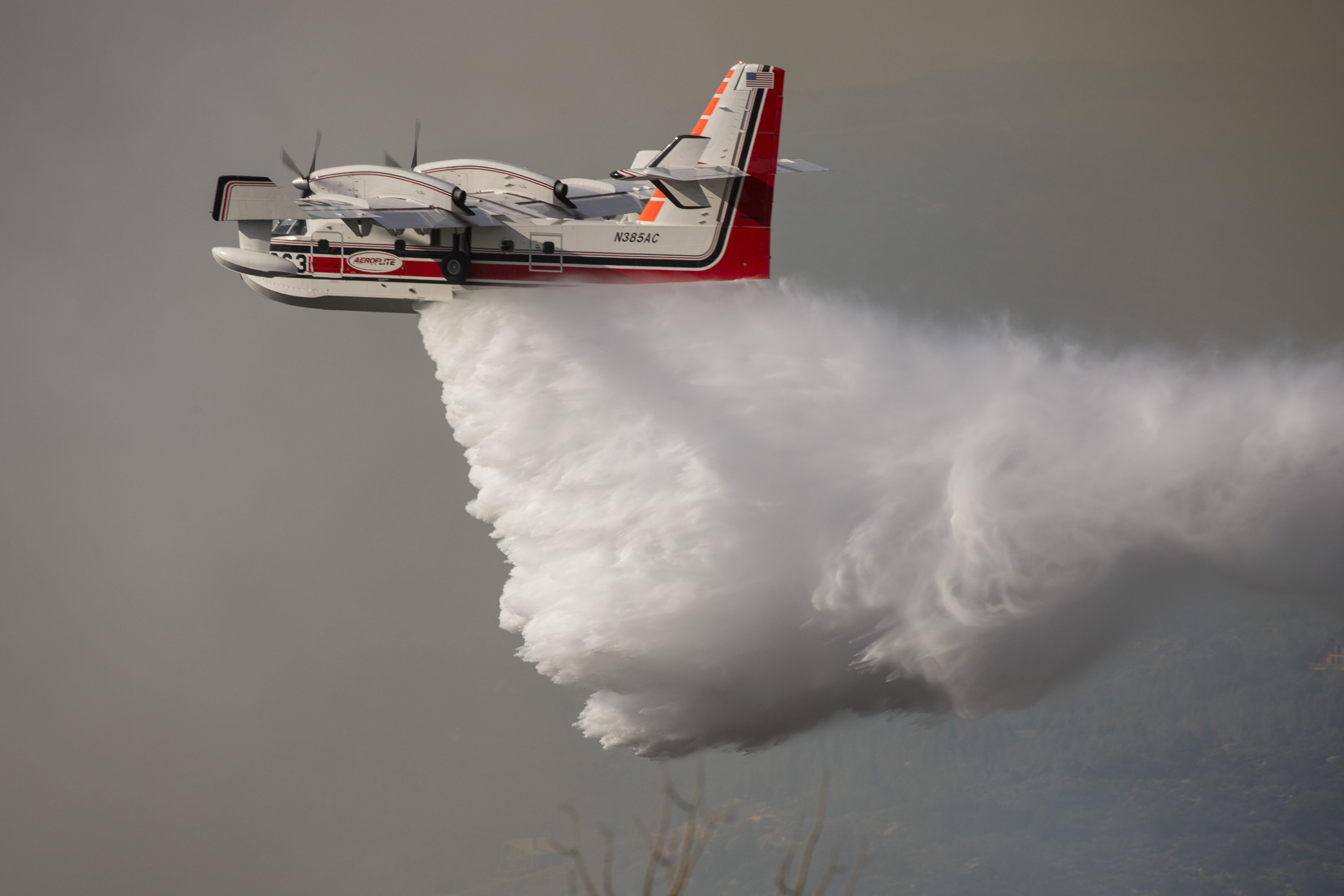In this image, a specialized firefighting aircraft is captured mid-action in a hazy, foggy sky. Positioned in the upper left corner, the plane has a unique, rectangular body style distinct from typical aircraft. It's predominantly white with red accents; a striking red stripe runs through the middle and curves up the rear of the upright tail wing, while orange lines decorate the front of the tail wing and the rear section. The bottom of the plane is red, seamlessly transitioning to a white inset on the wings, which appear plastic-like and house bulky propeller bases. The propellers are prominently visible, with two at the front and a gray tip bordered in black completing the aircraft's nose. Below the plane, a voluminous cascade of water, resembling a white fluffy cloud, is being released, suggesting the plane is actively engaged in firefighting efforts. The background further enhances this narrative, with hazy gray skies obscuring specific details of the landscape, though faint hints of foliage and water are visible towards the bottom right, framing the scene of aerial firefighting.